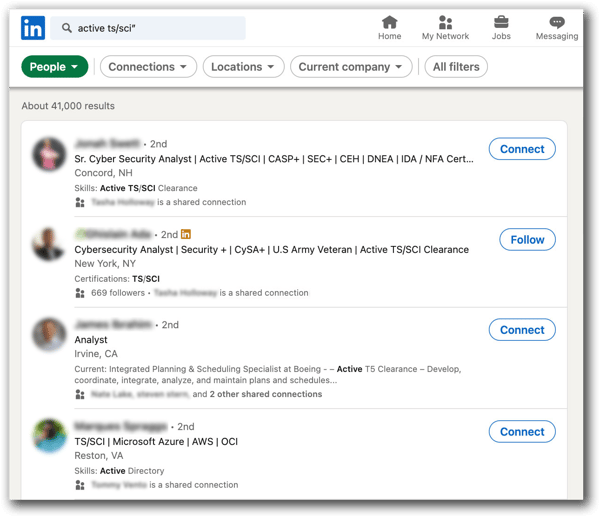This image depicts a detailed view of a LinkedIn webpage. At the very top, a light gray border frames the entire page. At the upper-left corner, there is a distinctive blue square featuring the LinkedIn logo ("IN"). Directly to its right, a search bar displays the text "Active TS/SCI" accompanied by a star icon.

Moving horizontally across the top navigation bar, the options "Home," "My Network," "Jobs," and "Messaging" are clearly visible. Below this, there is a secondary navigation menu including "People," "Connections," "Locations," "Current Company," and "All Filters," each with respective drop-down menus apart from "All Filters." Notably, the "People" category has a green background with white text.

Descending further down the page, there is a taupe-gray shaded section stating "About 41,000 Results." Here, the user profiles come into focus, albeit with names and profile images blurred out. The profiles offer details on each person's location, qualifications, and brief bios.

On either side of each user profile are action buttons labeled "Connect" and "Follow," highlighted with blue outlines and blue text. This well-organized layout and color scheme enhance the information's clarity and ease of navigation.